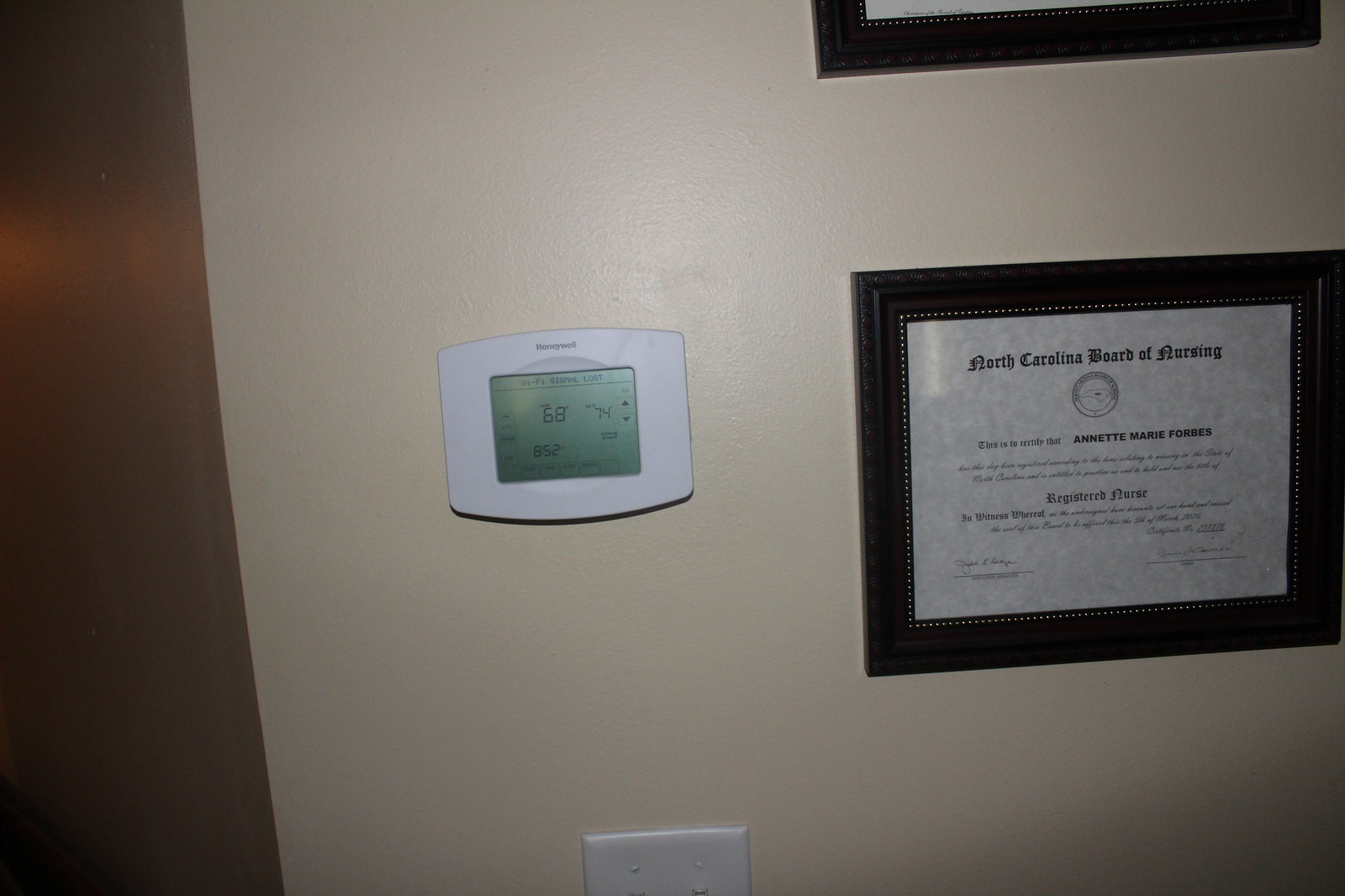In the photograph, a beige-colored wall serves as the background. To the left side of the wall, there's a partially visible wooden door. Centrally located on the wall is a digital thermostat by Honeywell, which displays the time as 8:52 and indicates the current indoor temperature as 69°F, while the desired temperature is set to 74°F. Below the thermostat, in the middle of the image, a white plastic wall plate with an electrical outlet is visible. To the right of the thermostat, a framed diploma is prominently displayed. This diploma, awarded to Annette Marie Forbes by the North Carolina Board of Nursing, certifies her as a registered nurse. The diploma is enclosed in a black wooden frame with intricate beading and covered with glass, reflecting ambient light. The document itself is printed on gray parchment, featuring the logo of the North Carolina Board of Nursing.